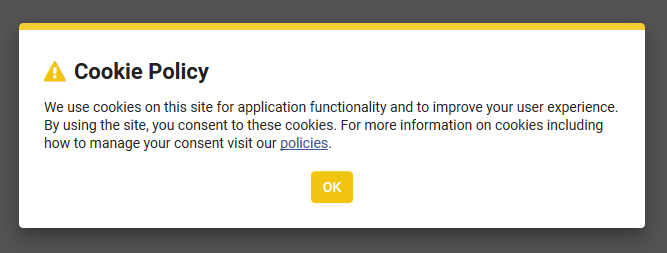The image features a rectangular border in gray. Inside this border is a white rectangle that occupies most of the space. Across the top of the white rectangle is an orange stripe, followed by an orange-yellow triangle underneath it. The triangle contains a white exclamation point. Below these elements, bold black text reads, "Cookie Policy."

Following this header, a smaller black font provides the message:
"We use cookies on this site for application functionality and to improve your user experience. By using the site, you consent to these cookies. For more information on cookies, including how to manage your consent, visit our policies."

The word "policies" is blue, underlined, and clickable, as is the blue period following it.

At the bottom right corner of the rectangle, there's a gray button with a white border that has the word "OK" in white text centered within it. This button has an Amish box style outline. The text "Cookie Policy" is not only the largest and boldest but also serves as the main header of the notification. The rest of the text, except for the blue "policies," is in a standard, unbolded black font.